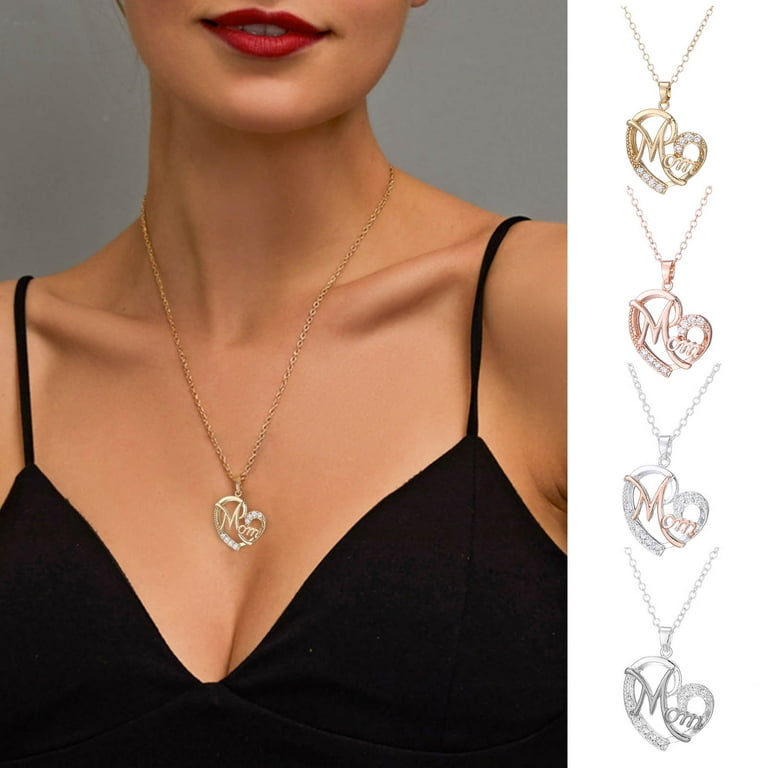This image is an advertisement for necklaces, likely intended for Mother's Day. The main area of the image, covering about three-quarters of the space on the left, features a photograph of a woman shown from just below her breasts to right below her nose. She is wearing a black, strappy top with a deep v-neckline and red lipstick, her collarbones prominently visible due to her slender frame. Around her neck is a delicate gold chain necklace with a heart-shaped pendant that has the word "Mom" inscribed at its center.

On the right side of the image, there are four different versions of the same necklace displayed vertically. The variations include a full gold version, a rose gold version, a silver version with rose gold text, and a full silver version. These pendants, similar in design to the one worn by the woman, feature heart shapes with "Mom" inscribed at their centers and small jewels adorning the edges. The detailed portrayal of these necklaces highlights the different material options available for this heartfelt piece of jewelry.